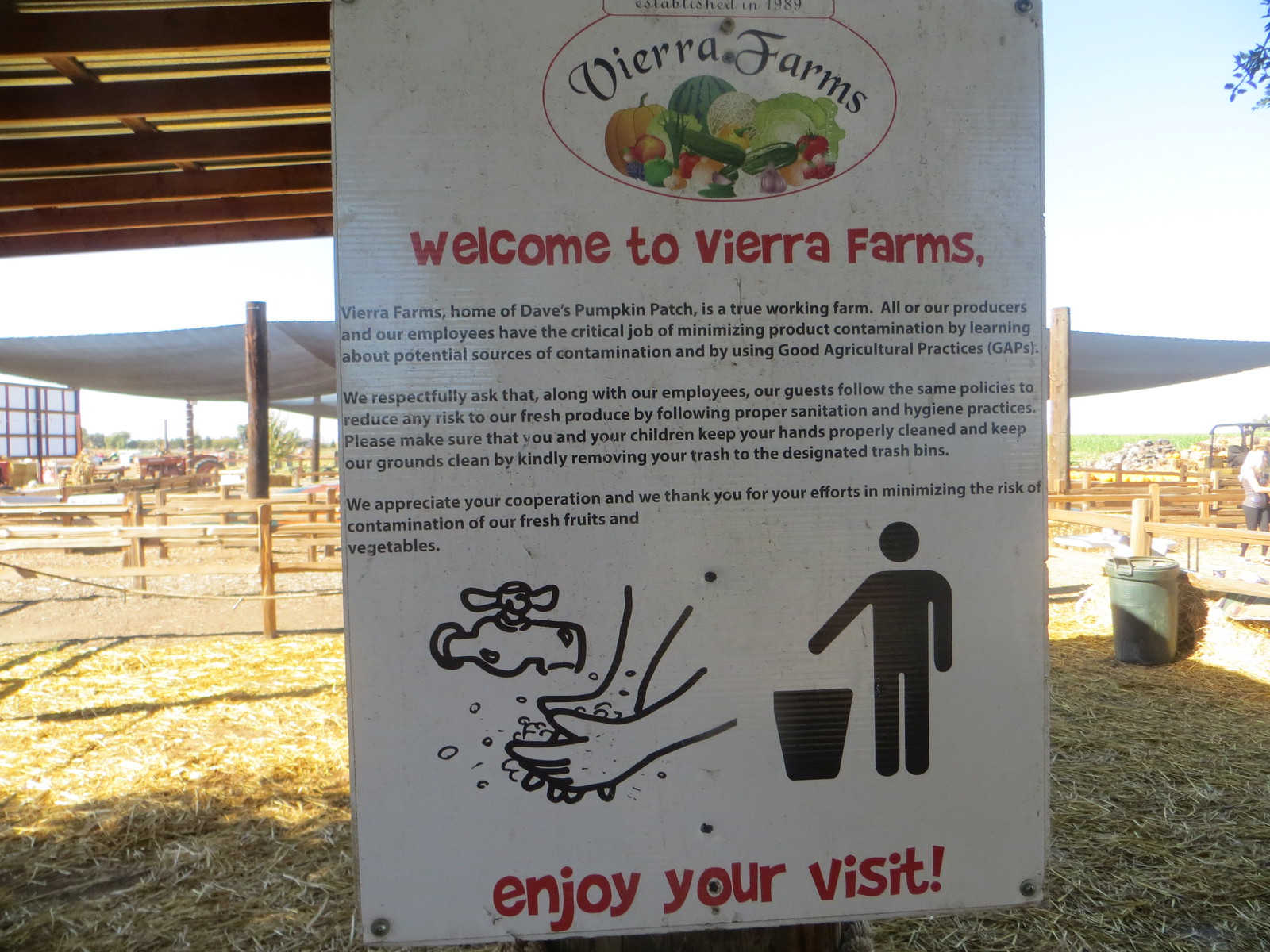The sign, mounted on a post in an outdoor farm setting, features essential information for visitors. The white sign, although slightly dirty, prominently displays "Vieira Farms" at the top within an oval. Below that, a colorful illustration of various vegetables appears, followed by the red-lettered welcome message: "Welcome to Vieira Farms." It reads, "Vieira Farms, home of Dave's Pumpkin Patch, is a true working farm. All of our producers and employees have the critical job of minimizing product contamination by learning about potential sources of contamination and using good agricultural practices (GAPs)."

Further down, the sign explains that guests are expected to follow the same sanitation and hygiene practices to keep hands clean and dispose of trash properly, in designated bins, to help reduce the risk of contamination of fresh produce. The bottom portion includes line drawings; one shows a faucet with hands being washed, and another depicts a person discarding litter into a trash can. The sign concludes with "Enjoy your visit!" and expresses appreciation for visitors' cooperation in maintaining cleanliness.

The backdrop features hay scattered on either side, wooden corrals with coverings, a large trash can, and a person visible on the right side, emphasizing the active farm environment. The sign, accented with colors like red, green, orange, black, and purple, serves as a detailed guide for guests on proper hygiene and cleanliness practices while visiting the farm.